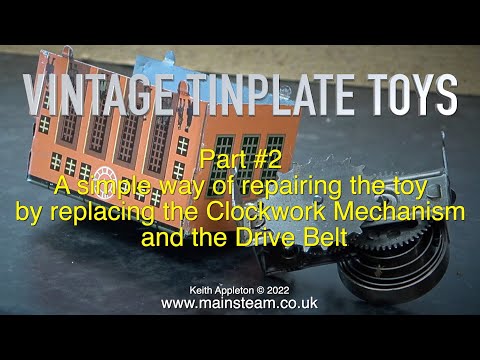The image features a vintage tin plate toy displayed in an indoor setting, accompanied by detailed informational text. The prominently displayed text at the top of the image reads "Vintage Tin Plate Toys" in white, followed by "Part Two: A Simple Way of Repairing the Toy by Replacing the Clockwork Mechanism and the Drive Belt." Below this text, there's a close-up of the toy, which resembles a peach-colored, house-like structure with long rectangular windows framed in brown and gray trims. The toy is connected to a set of gears and a large spring mechanism, visible in the foreground, suggesting the inner workings of the toy. Additional text at the bottom of the image includes the notation "Keith Appleton, copyright 2022, www.mainstream.co.uk" in white letters. The background features an image of another tin toy resembling a camera on a turntable, giving further context to the main subject.